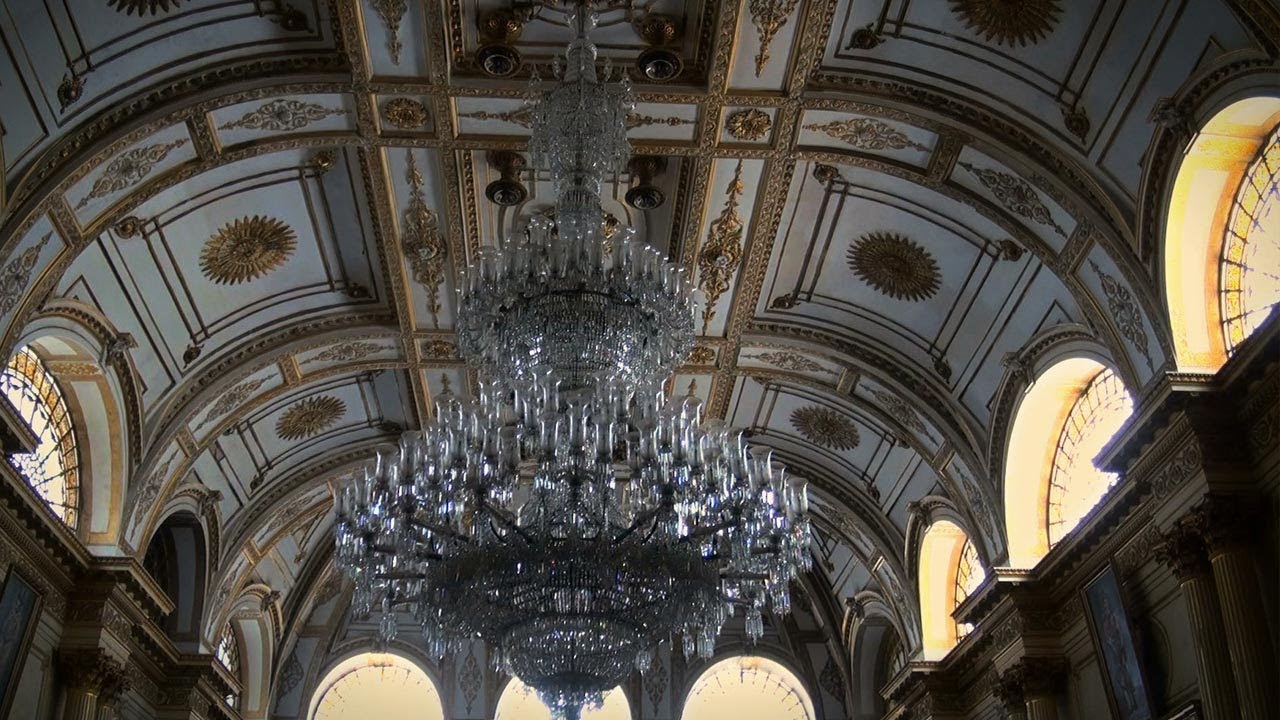In the image, there is a grand room featuring an elaborate chandelier suspended from a remarkably high ceiling, approximately 30 feet up. The ceiling itself is curved and decorated with intricate white and gold patterns, including sun-shaped designs and large, rectangular panels adorned with gold trim. Surrounding the ceiling, half-moon stained glass windows allow natural light to filter through, and these windows are positioned where the walls meet the ceiling.

The chandelier is the centerpiece of the room, massive and intricate, likely 10 to 12 feet in height. It consists of three concentric circles, with the largest at the bottom and the smallest at the top. Each circle is crafted with thick glass on the exterior and thinner glass pieces within, all adorned with clear glass jewels. Numerous bulbs, resembling tall, clear glass elements, are attached to the thick parts of each circle, directed upwards. The chandelier's sheer complexity and heavy appearance underscore its luxurious nature, suggesting that a significant amount of money was invested in its creation.